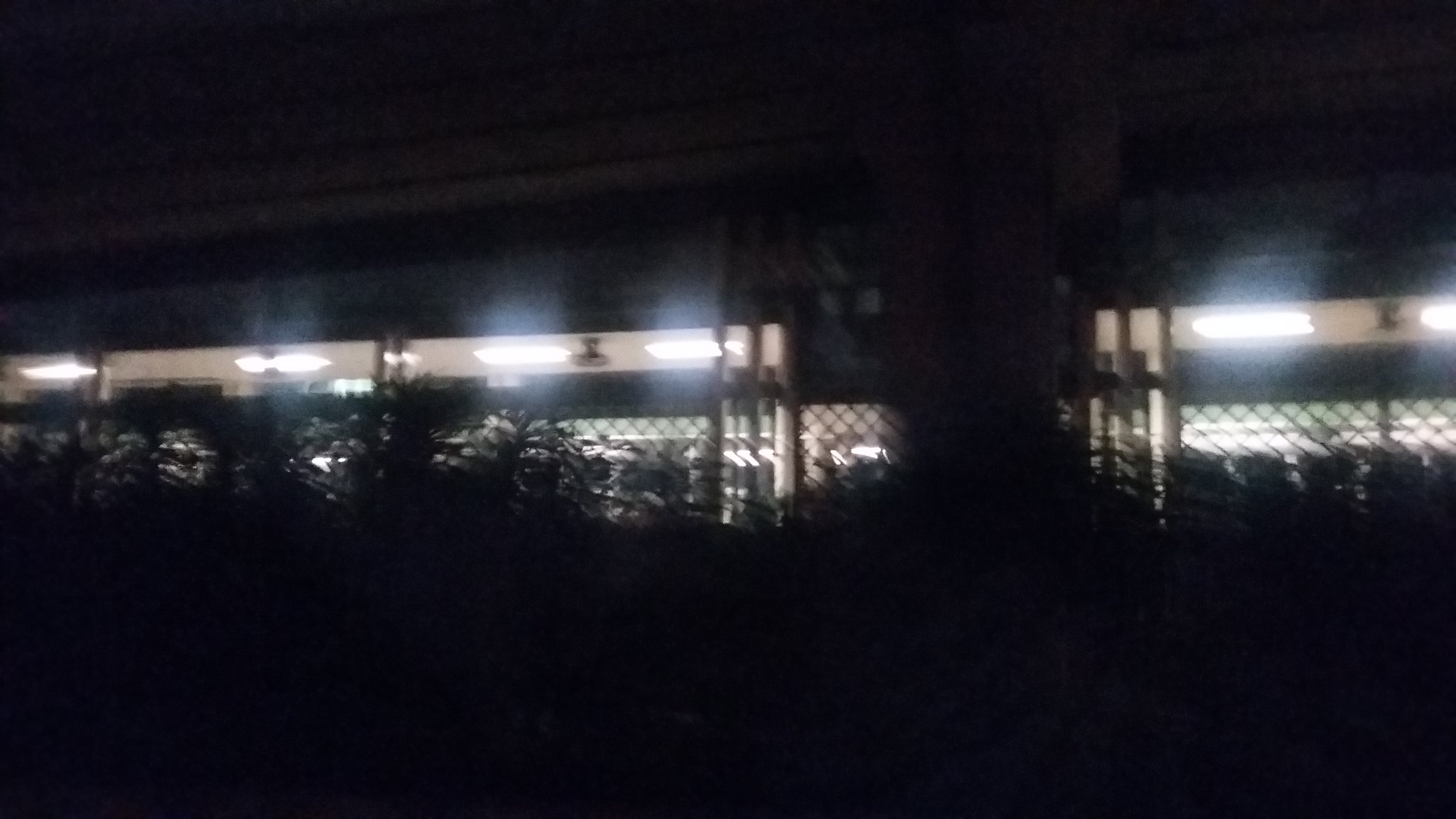This nighttime photograph captures a dark, enclosed area that appears to be located in the back of a store or a warehouse. The scene is dominated by very bright, evenly spaced fluorescent lights suspended above multiple sections divided by chain-link fencing. These barriers feature pillars and hide behind them what could be stacks of products, possibly gardening supplies, as suggested by the presence of trees or bushes along the foreground, obscuring parts of the fence. The bright lights illuminate this warehouse-like area, revealing a repetitive pattern that extends from the right to the left side of the image, with a black hallway visible between the enclosed sections. The overall ambience is shadowy with strong contrasts due to the intense lighting against the dark surroundings.